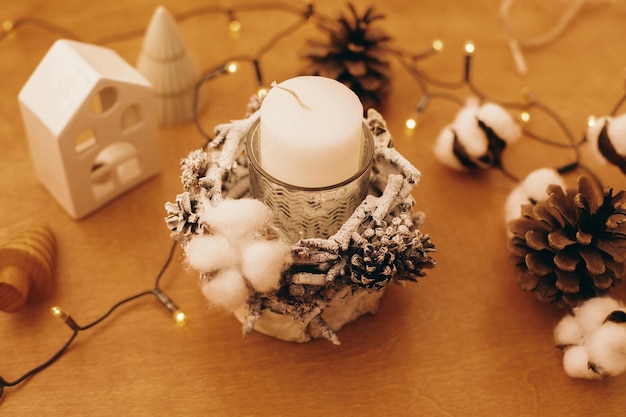The image captures a charming holiday art scene on a light brown wooden table, elegantly decorated for the winter season, most likely Christmas. Central to the composition is a handcrafted candle holder adorned with pine cones, bits of cotton, and a sprinkling of artificial snow, cradling an unlit white candle in a silver glass holder. Interwoven through this cozy setting are golden Christmas lights, casting a warm glow. To the top left, there's a small white house with an adjacent white Christmas tree, while nearby, a wooden toy adds a playful touch. Scattered around are additional pine cones and tufts of cotton, enhancing the festive and rustic ambiance of the display.